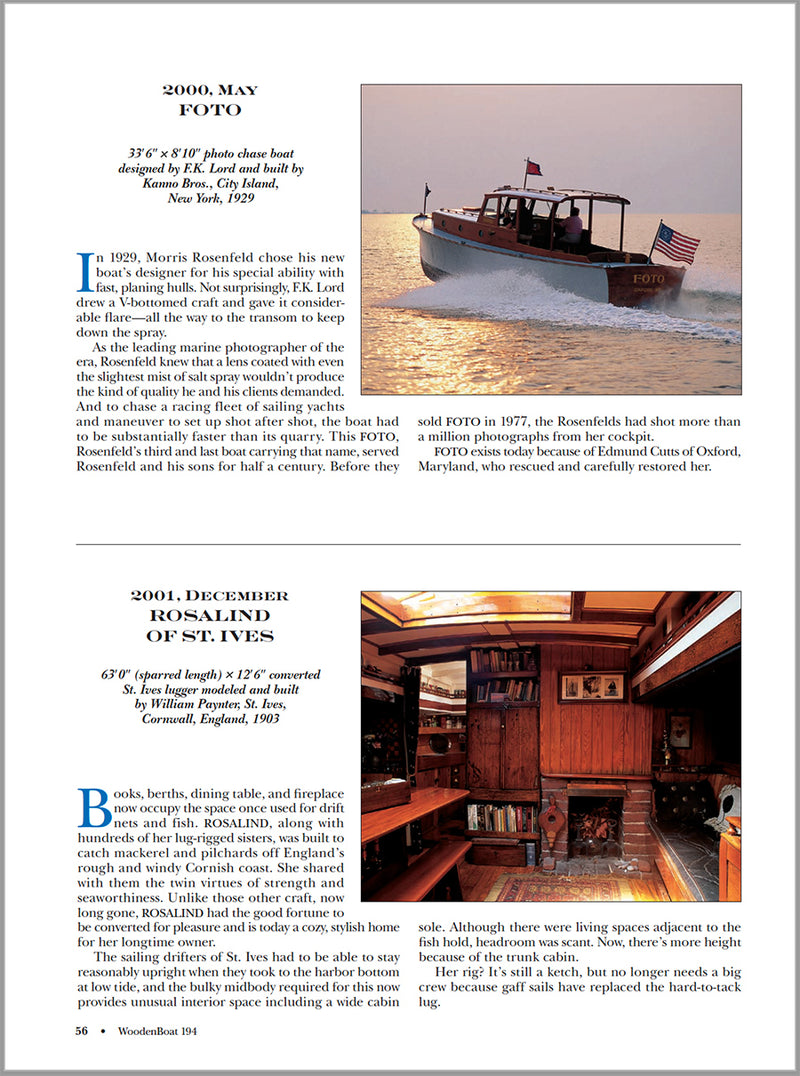The image is a print advertisement featuring two distinct sections, both surrounded by text and edged in silver. The upper portion of the advertisement highlights a vintage 1920s wooden chase boat. This boat, identified by its name "FOTO" inscribed on its stern, also prominently displays an American flag on the bow and another flag on the cabin. The boat, described as designed by FK Lord and constructed by Kenzo Brothers in 1929, is depicted creating a white wake as it sails at sea, with two men visible on board. The photograph is labeled "2000 May FOTO Photo."

The bottom section of the advertisement shifts focus to the interior of a different boat, showcasing a more homely and intricate setting. The photograph reveals a cramped but cozy space featuring wooden panels, a mantel above a fireplace, bookshelves, a galley, and a built-in seating area with a wooden table and bench. This image is associated with the headline "2001 December Rosalind of St. Ives" and describes a vessel reportedly built in 1903. Both sections are accompanied by detailed narratives that further elaborate on the features and histories of the respective boats.